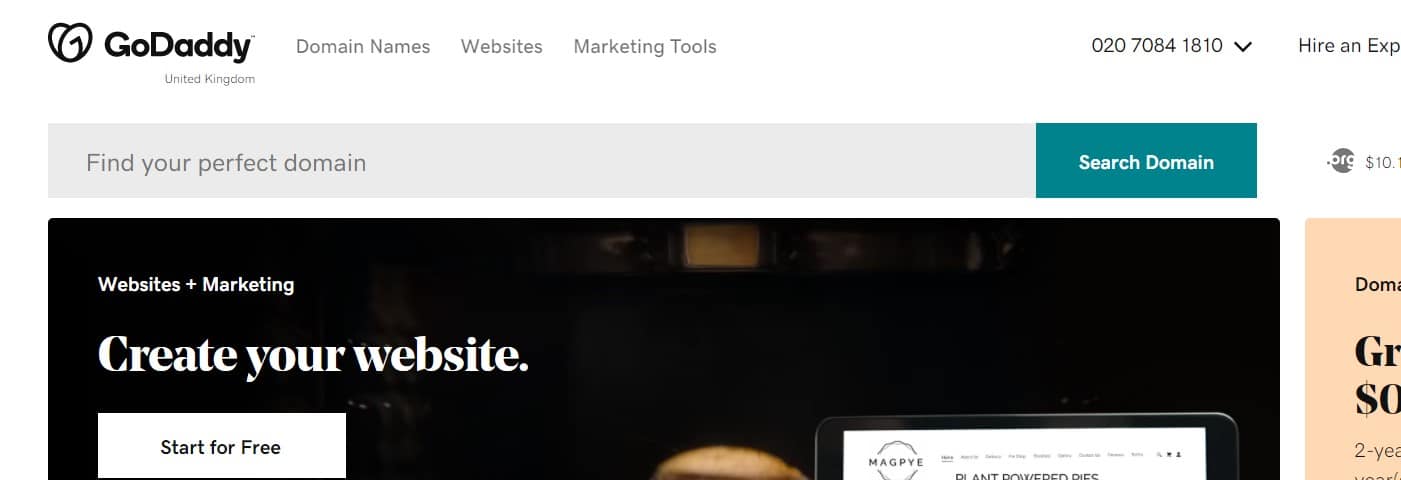The screenshot captures the top portion of a partially loaded web page, prominently featuring GoDaddy’s branding and service offerings. The page is framed by a black header housing a heart-like symbol followed by the bold black text "GoDaddy." Below that, in gray text, it mentions "United Kingdom."

To the right, the navigation menu includes links for "Domain Names," "Websites," and "Marketing Tools." A contact phone number, "020 7084 1810," is displayed with a down arrow indicating a dropdown menu. Just below, there's a call-to-action link, “Hire an Expert,” which uses capital letters for the H and E in "Hire an Expert."

The main content area begins with a gray bezel containing the instruction, “Find your perfect domain,” set against a dark gray background. To its right is a teal button with white text reading "Search Domain."

Further to the right, there is a black circle with "ORG" inscribed in white, accompanied by a dollar sign and the partial text "$10," although it is cut off.

On the left side, a section with a black background highlights the "Websites + Marketing" service. Bold white text urges users to "Create your website." Below, a white rectangle with black text offers a promotional button "Start for Free."

Additionally, on the right side, a partially visible mock-up shows the name "MAGPYE" with a hexagonal outline, both in a muted purplish hue. The background features shades of gold or brown, adding a touch of elegance to the design.